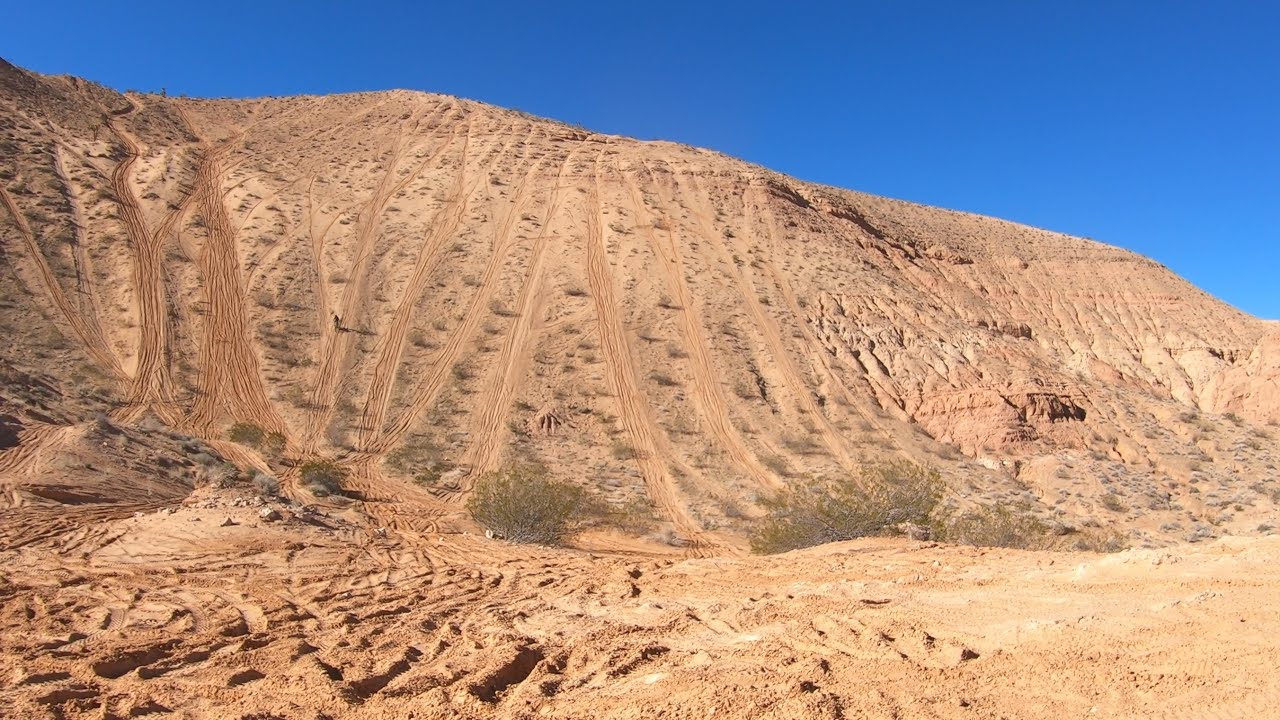In this vibrant outdoor photograph taken on a clear, bright day, the rich blue sky serves as a striking backdrop for a tall, sandy hill that dominates the scene. Captured from the perspective of someone looking up at the imposing hill, the image highlights the arid, dusty surroundings. Tire treads from two-wheeled vehicles, such as motorbikes and dirt bikes, crisscross the hill, indicating its use for off-roading activities. The base of the hill features a few dry bushes, while smaller, sparse brush continues halfway up the slope. Although some descriptions suggest the presence of a person on a motorcycle halfway up the hill, a closer inspection reveals no individual or vehicle in sight. The overall setting is desolate, with minimal vegetation and an undeniably arid atmosphere, painting a vivid picture of a remote and rugged terrain.